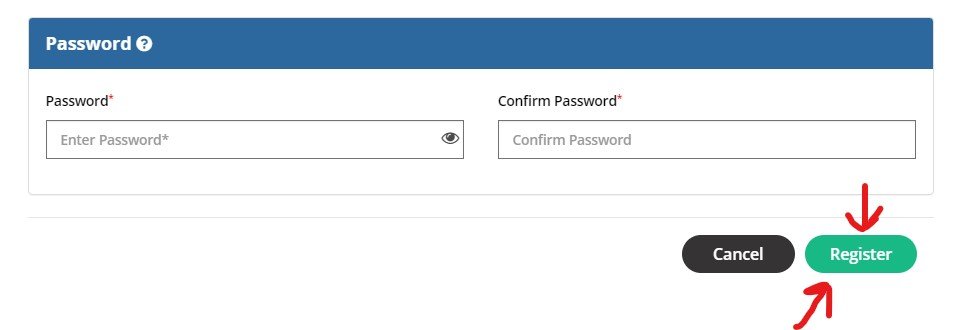This is a detailed screenshot of a password setup screen. At the top, a blue bar spans the width of the screen, featuring white text that reads "Password" on the left side, accompanied by a question mark icon. Below this blue bar, the background switches to white. There are two fields placed side by side: the left field is labeled "Password" and the right field is labeled "Confirm Password." Inside the left field, placeholder text reads "Enter Password," with an eye icon situated on the right side of the field, hinting at a show/hide password feature. The right field contains the text "Confirm Password."

Beneath these fields, two pill-shaped buttons are aligned horizontally. The "Cancel" button, which is black, resides on the left, and the "Register" button, which is green, is on the right. Notably, two red arrows are drawn on the screen: the first one above the "Register" button, pointing downward at it, and the second one below the "Register" button, pointing upward.

The entire setup is displayed against a white background, creating a clean and straightforward user interface for password entry and confirmation.